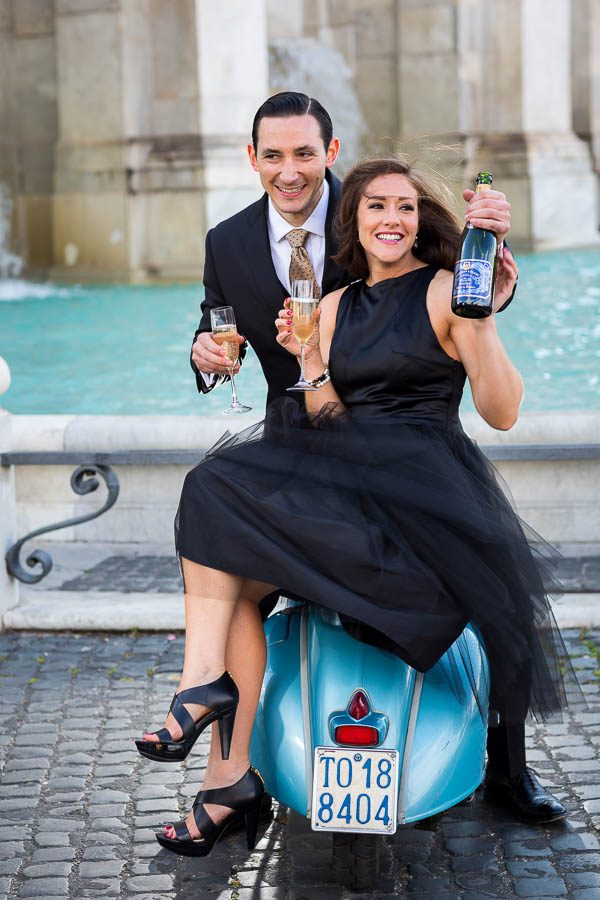In this tall, rectangular photograph, a cheerful man and woman are comfortably seated on a blue Vespa-style scooter, boasting the license plate T0188404. The woman, dressed in a sleeveless black dress and black sandal heels, sits at the front with her head turned slightly right, raising a champagne glass filled with a yellow liquid. Her legs dangle to the scooter’s left side. Behind her, a smiling man with slicked-back black hair sports a black suit, white shirt, and a gold tie with dots. He holds a champagne bottle over the woman’s shoulder. This joyful scene is set before a blue concrete fountain, surrounded by a square gray stone ground.